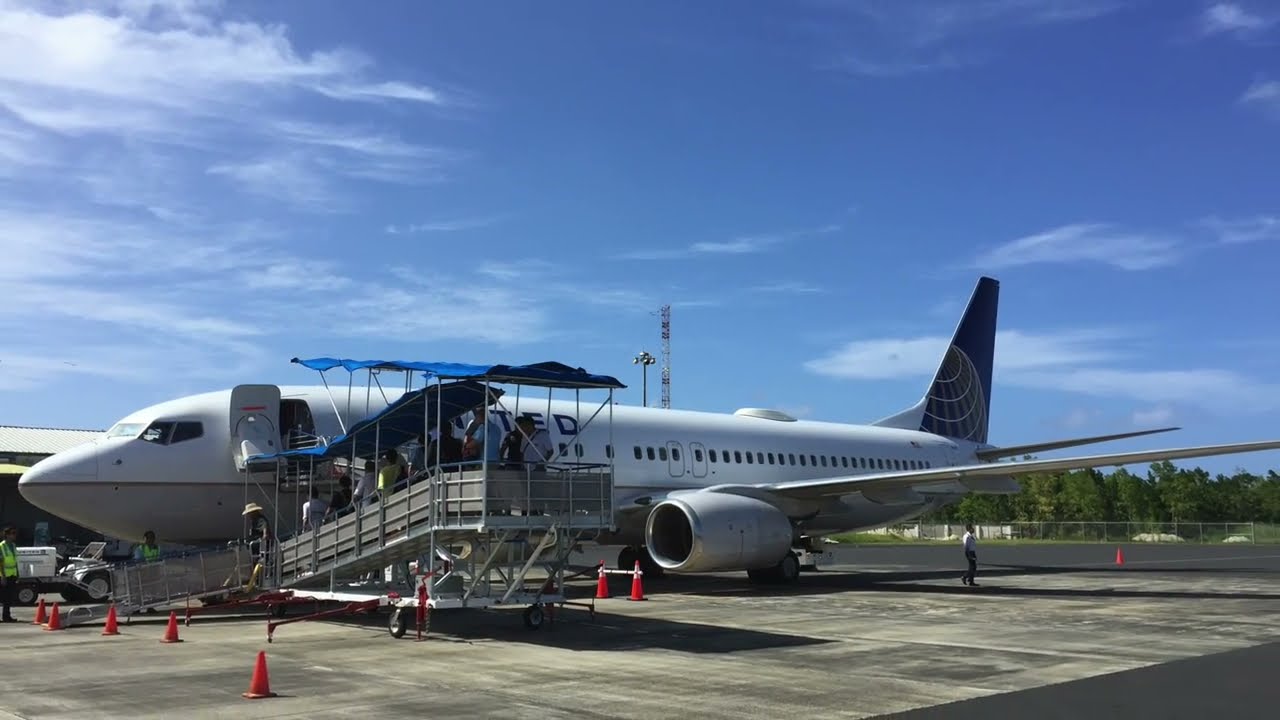This photograph captures a portion of an airstrip from the perspective of a passenger looking out the right side of a plane. Dominating the lower right quadrant of the image is the front part of a white airplane, specifically highlighting its right wing, which features a partially blue vertical stabilizer. The plane casts a shadow onto the brown pavement of the runway below. Adjacent to the runway, the fenced-in area is plain with patches of weeds and grass, some areas appearing dry and barren. Beyond the fence, there's a lush green field and a dense area of trees. In the background, a tall hill or mountainous terrain rises up, set against a mostly clear blue sky with a few white, puffy clouds. The image also shows periodically spaced light poles and some circular painted markings on the pavement with something sticking up, possibly a light. The main colors in the photograph are green, white, and blue. Notably, there are no people or text visible in the scene.